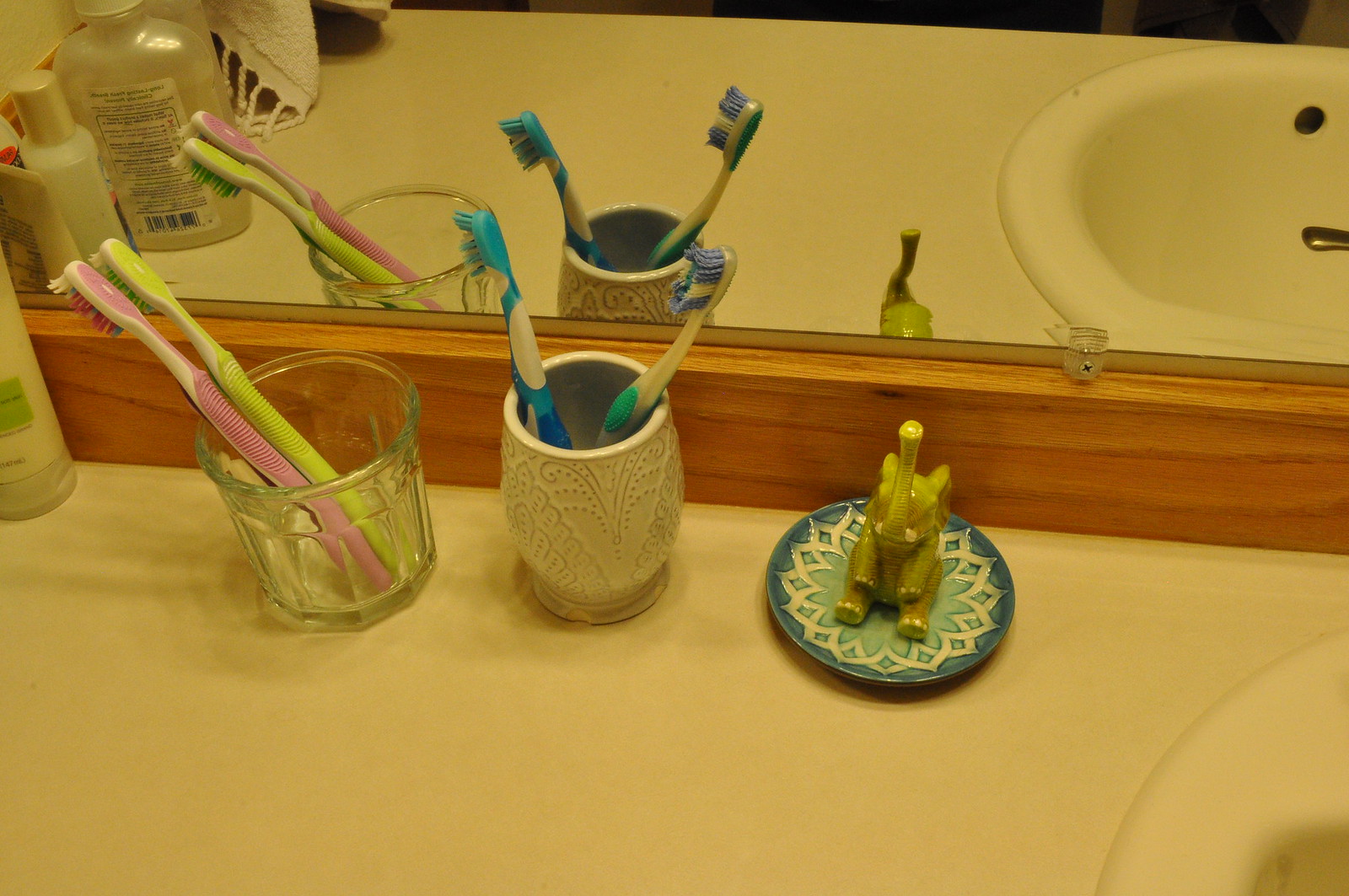The image captures a close-up view of various objects arranged on a bathroom counter, with a mirror in the background reflecting the scene. On the far left, there is a glimpse of a bottle of lotion. Adjacent to the lotion is a transparent glass cup containing a pink paintbrush and a lime green paintbrush. Next to this is a white porcelain cup holding two toothbrushes: one is light blue with white stripes, and the other is dark blue with white patterns. Further along the counter, there's a small, colorful dish with a flower pattern, featuring a gold elephant figurine with its trunk up. In the very bottom right corner, part of a round sink is visible. The mirror reflects all these items, as well as additional containers of soaps and other bathroom products positioned on the left side of the counter, adding depth and context to the bathroom setup.